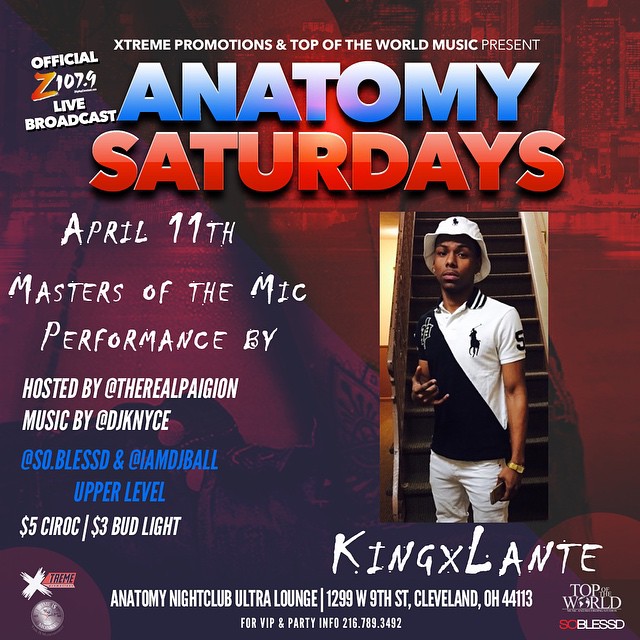This promotional flyer, set against a vibrant red and purple, grungy background, advertises "Anatomy Saturdays," presented by Extreme Promotions and Top of the World Music. The top left corner proudly features "Official Z107.9 Live Broadcast." Centrally displayed at the top, bold text announces "Extreme Promotions and Top of the World Music Present" with "Anatomy Saturdays" in prominent blue and red lettering across the flyer.

Scheduled for April 11th, the event promises a "Masters of the Mic Performance," taking place at Autonomy Nightclub Ultra Lounge, located at 1299 West 9th Street, Cleveland, OH 44113. For additional VIP and party information, guests can contact 216-789-3492. 

The lineup includes lively performances hosted by The Real Pherealpai John (spelled T-H-E-R-E-A-L-P-A-I-G-I-O-N) and featuring music by DJKNYCE, So Blessed, and IMDJPAW. On the left, the flyer highlights $5.00 Ciroc and $3.00 Bud Light specials for the upper level.

The right side of the flyer showcases a man identified as King Exalante (spelled K-I-N-G-X-L-A-N-T-E), presumably the lead performer. He is depicted wearing a distinctive black and white polo shirt, split from the shoulder down, paired with a white cap, and stands in front of a flight of stairs, adding a casual yet stylish touch to the overall design.